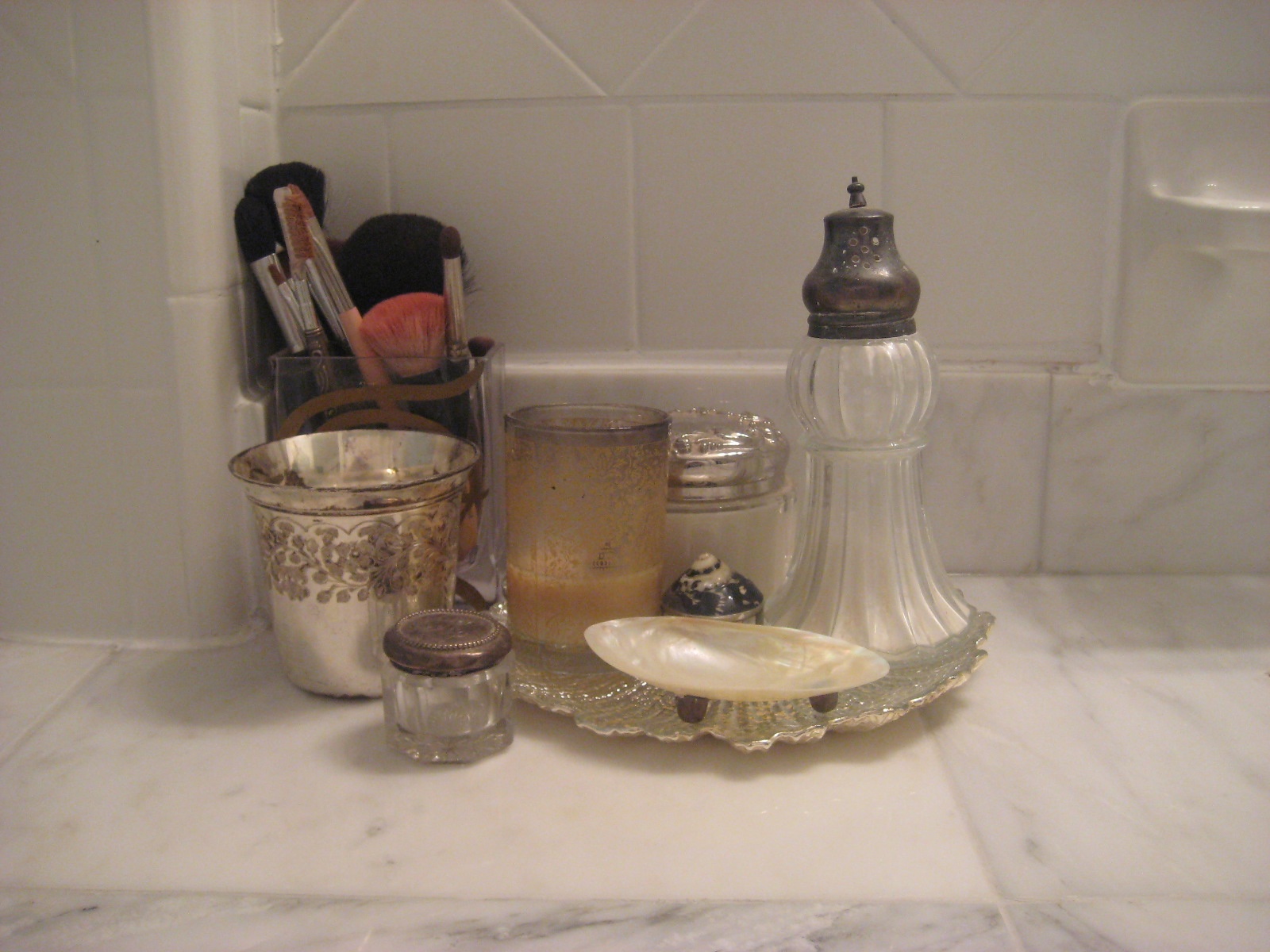In this photograph, we observe a neatly arranged bathroom countertop. The counter surface is a shiny gray material, complementing the grayish-white tiles of the backsplash. Centered on the countertop is a sleek silver tray that holds a variety of bathroom items, enhancing the overall aesthetic.

On the tray sits an open seashell soap dish, ideal for a small bar of soap. Beside the dish is a glass candle holder, with the candle burned down to its lower fourth and colored a deep brown. The rim of the candle holder is blackened from previous use, indicating it has been frequently lit.

To the left, there is a silver decorative cup with intricate engravings around its edge. This cup appears to serve as a rinsing glass, likely used during daily oral hygiene routines. Leaning against the tile wall is a square plastic container filled with a variety of makeup brushes. These brushes have handles ranging from skinny to thick, with bristles mostly black except for one brush with striking pink bristles.

In the upper right corner of the image, part of a wall attachment is visible, designed to hold a toothbrush. Notably, it is currently empty, adding a touch of minimalism to the scene.